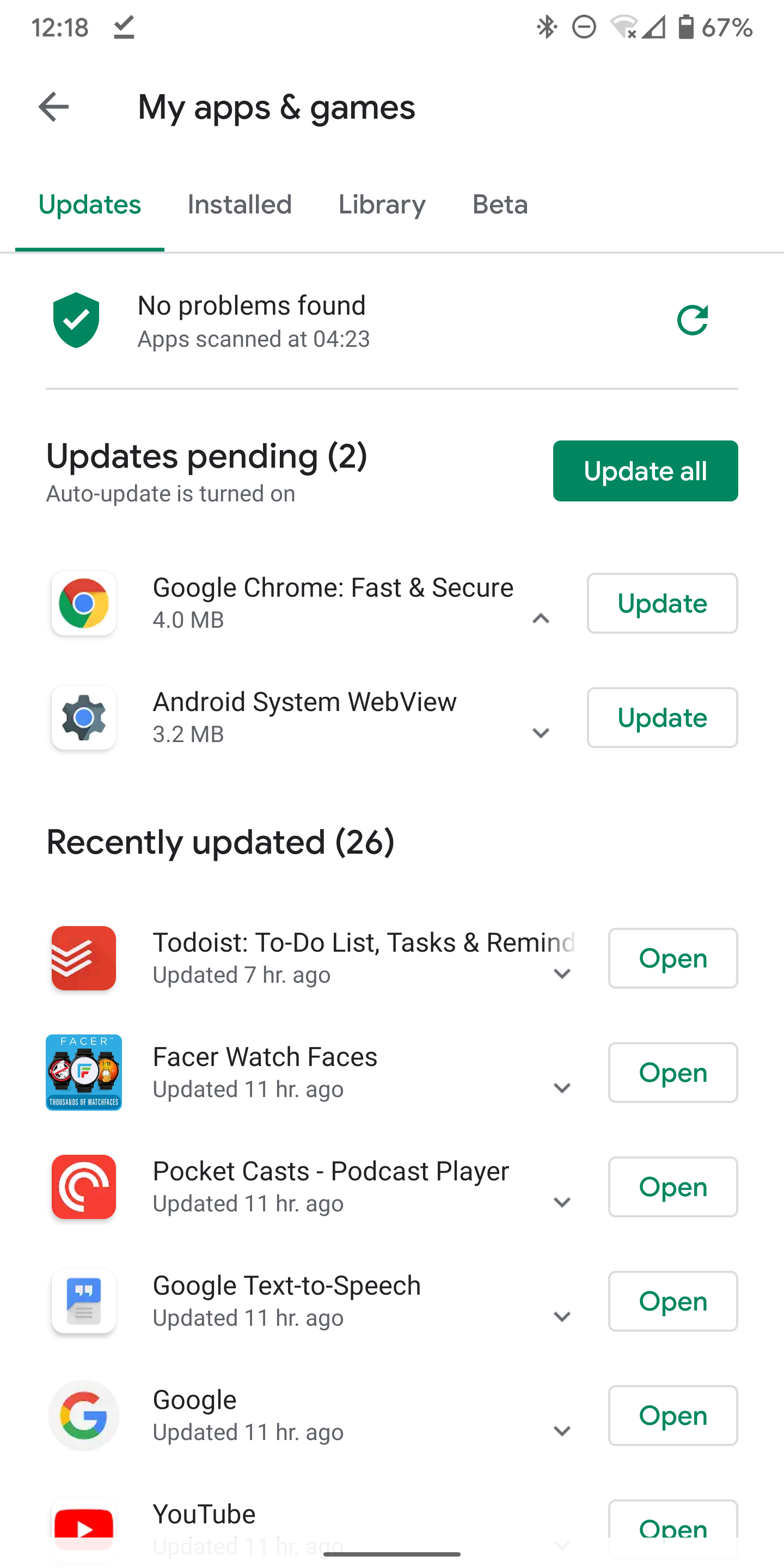The image depicts a smartphone screen showcasing various app updates and system notifications. The screen displays several key pieces of information, including the current battery percentage at 67%, active Bluetooth and Wi-Fi connections, and an indication that there are 432 updates pending with auto-update enabled.

Here's a detailed breakdown of the updates listed:

1. **Google Chrome**:
   - Description: Fast and secure web browser.
   - Update Size: 4 megabytes.

2. **Android System WebView**:
   - Update Size: 3.2 megabytes.

3. **Recently Updated Apps**:
   - **To-Do List, Tasks, and Reminders**:
     - Last Updated: 7 hours ago.
   - **Watch Faces App for Smartwatches**:
     - Last Updated: 11 hours ago.
   - **Pocket Casts Podcast Player**:
     - Last Updated: 11 hours ago.
   - **Google Text-to-Speech**:
     - Last Updated: 11 hours ago.
   - **Google Services**:
     - Last Updated: 11 hours ago.

4. **YouTube**:
   - Multiple instances of 'Open' and 'Update' options appear, suggesting either a glitch or multiple pending actions for this app.

The phone indicates that the device is performing an app scan, with no problems found, and that updates are installed periodically by the system. The image gives an overview of app management on an Android device, highlighting the efficiency of modern app updating processes, and showcases the essential information a user might need to navigate their device's software updates.